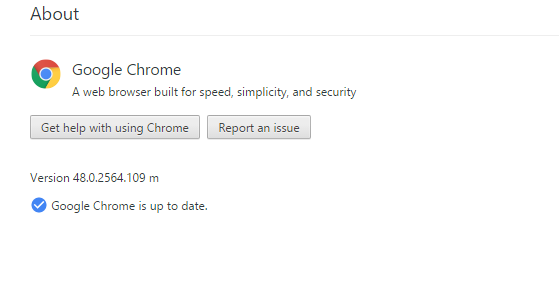The website features a minimalist design, dominated by a clean white background. At the top, a thin black line traverses from the left to the right, subtly accentuating the upper boundary of the page. Below this line, the word "About" is prominently displayed. Further down, a large, vivid Google Chrome logo, showcasing its iconic red, green, blue, and yellow colors, serves as the focal point.

Beneath the logo, a concise tagline reads: "A web browser built for speed, simplicity, and security." Directly below the tagline is a light gray navigation bar offering two options: "Get help with using Chrome," available for additional user support, and "Report an issue," for submitting feedback or bugs.

The page specifies the browser version as 48.0.2564.109m, along with a reassuring message that "Google Chrome is up-to-date." This information is accompanied by a blue circle containing a white check mark, symbolizing that the browser is current.

The overall aesthetic is restrained and straightforward, emphasizing functionality and ease of navigation, with the colorful Chrome logo being the primary visual element against an otherwise stark, white background.